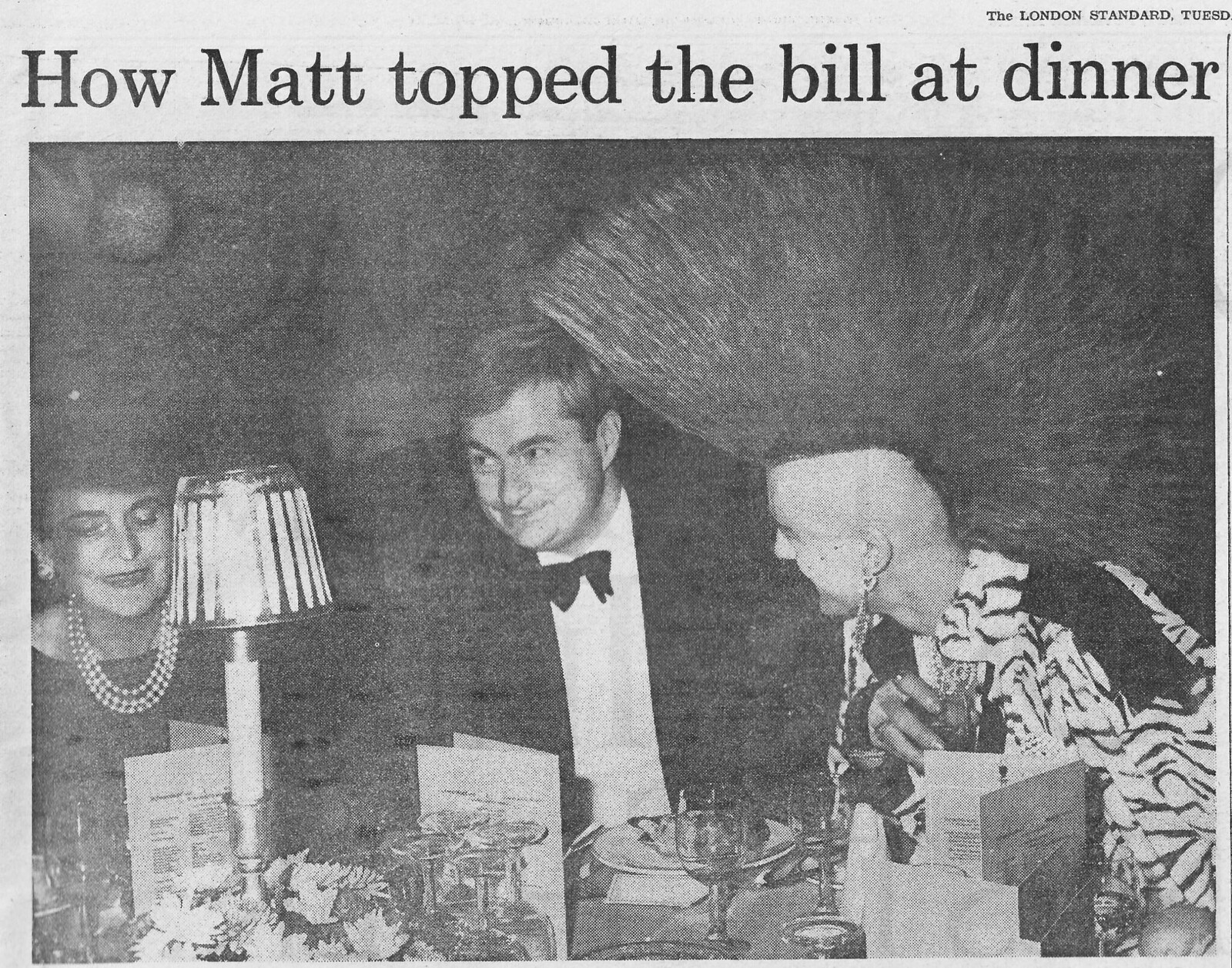The black-and-white photograph, likely from a newspaper, features a headline in bold black letters that reads, "How Matt Topped the Bill at Dinner," with a mention of "The London Standard Tuesday" in smaller print in the upper right corner on a gray backdrop. The image captures an elegant dinner scene with three individuals. On the left, a woman in a dark blouse adorned with pearls and beads gazes at a menu while sitting behind a lamp. The central figure, a smiling man, is dressed in a dark suit, white shirt, and bow tie. To the right, a striking figure wears a dramatic zebra-patterned jacket, complete with a towering Mohawk hairstyle and shaved sides. His outfit features wide black stripes on the shoulders and he holds a glass in his right hand. The table is cluttered with various glassware, emphasizing the sophisticated nature of the gathering.